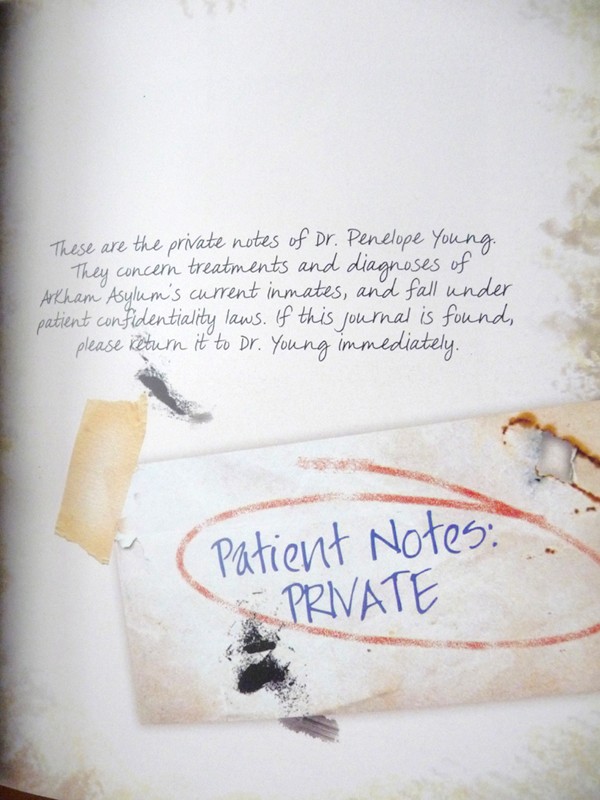This image appears to be a scanned page of a book, depicting a white piece of paper with detailed art and text. The page features a digitally created photograph that combines various textures and elements to mimic a realistic document. The central text, written in a dark gray or light black handwritten font, reads: "These are the private notes of Dr. Penelope Young. They concern treatments and diagnoses of Arkham Asylum's current inmates and fall under patient confidentiality laws. If this journal is found, please return it to Dr. Young immediately." This note occupies the center of the otherwise white page that exhibits staining textures around its edges. Attached to the main document is a burnt piece of paper, outlined in red marker or chalk, with the words "Patient Notes, Private" written in a blue semi-handwritten font. This paper looks slightly worn and torn, suggesting its aged appearance. The overall image seems to be a meticulously crafted item, likely related to a project within the Batman Arkham Asylum series.